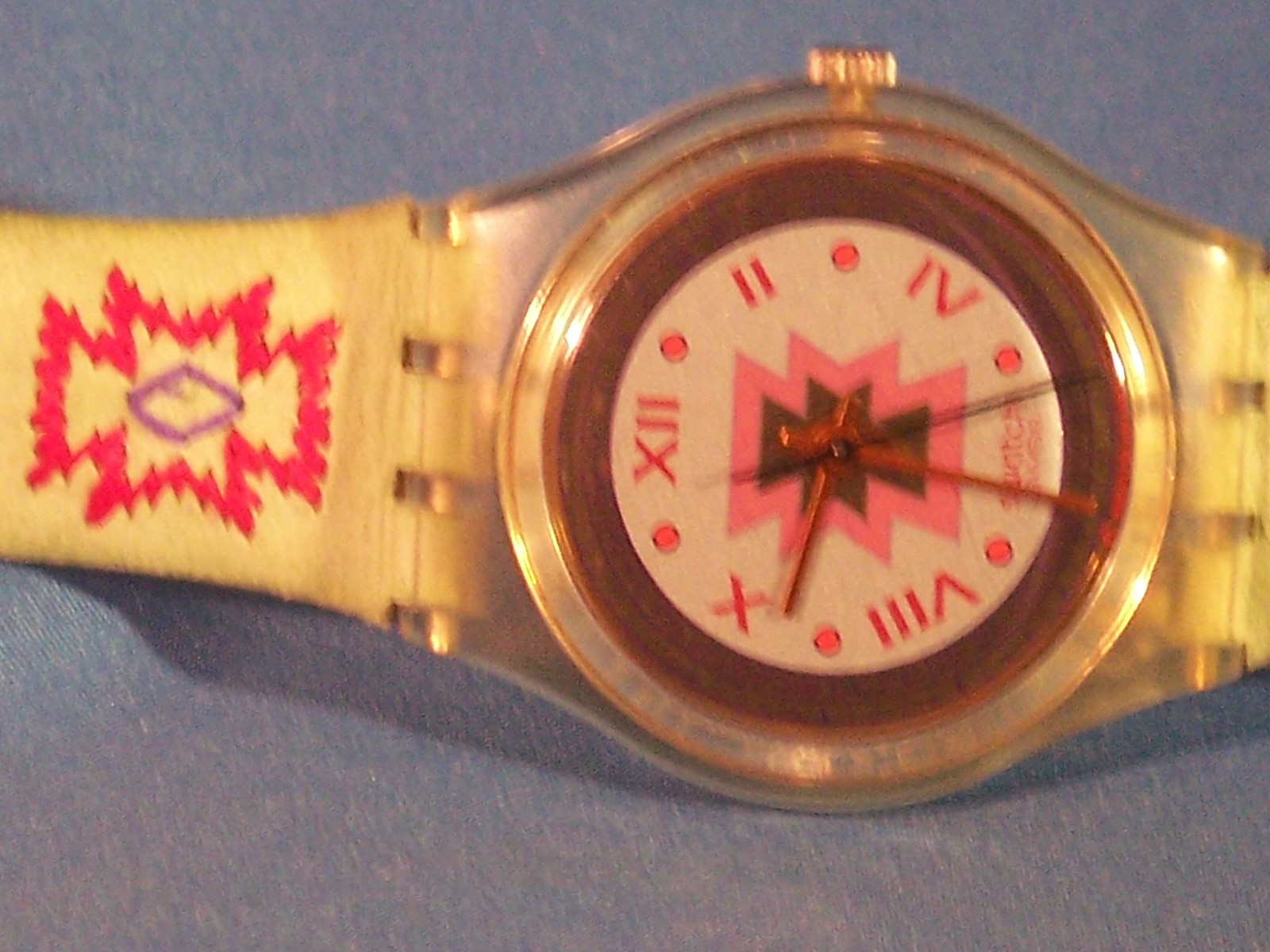This Swatch watch, likely from the 1980s, showcases a vibrant vintage aesthetic. Its design features predominantly plastic components, embodying the era's characteristic style. The timepiece is adorned with intricate tribal motifs that extend across both the dial and the strap. The watch face is highlighted by a bold red border which frames the tribal design, rendered in a blend of purple hues on the left side. Within the dial, a similar pattern in pink contrasts against a black interior, housing two distinct watch hands.

The unconventional numeral layout resembles Roman numerals interspersed with dots, contributing to its unique time-keeping display. The exterior of the strap stands out in a bright yellow, made from durable plastic, while the inner portion is fashioned from transparent material, offering a glimpse of the underlying mechanism. This juxtaposition of vivid colors and clear components exemplifies the innovative and playful design ethos of Swatch during that period.